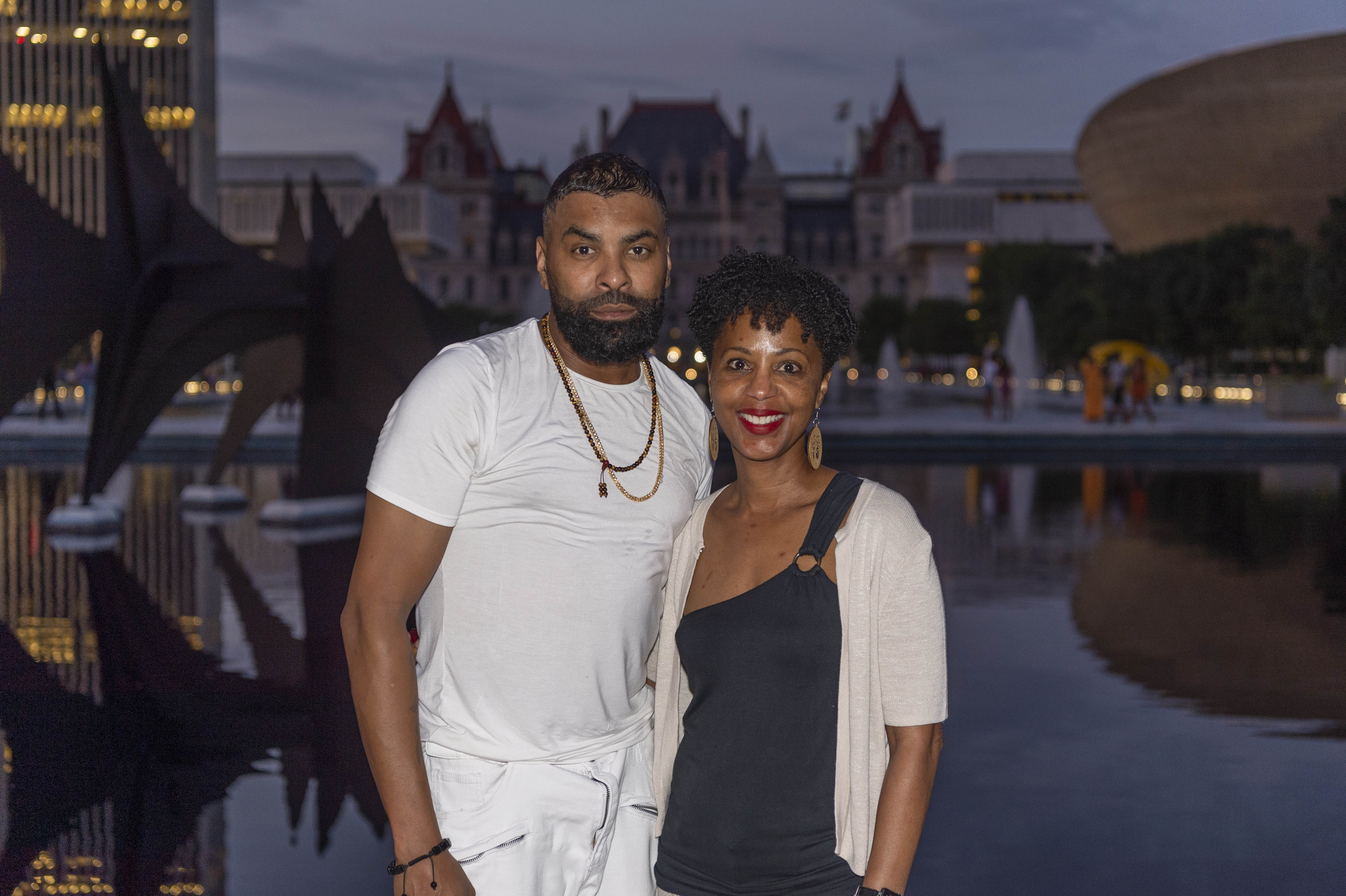In the foreground of the image, a shallow body of water covers the ground surface, reflecting the ambient light of the late evening. Several fountain structures are visible in the background, gracefully spraying water into the air. Scattered around the area are people leisurely walking, adding a dynamic touch to the serene setting. In the center of the image stand a man and a woman, both gazing directly at the camera, making them the focal point of the composition. Behind them, historical buildings rise into the background, creating a picturesque blend of architecture and landscape. Overhead, the dimming sky transitions through an array of colors, including black, white, brown, red, gold, tan, maroon, orange, and yellow, adding depth and warmth to the scene. This outdoor setting, captured in the mellow light of the late evening, draws attention to its historical charm and the tranquility of its surroundings.